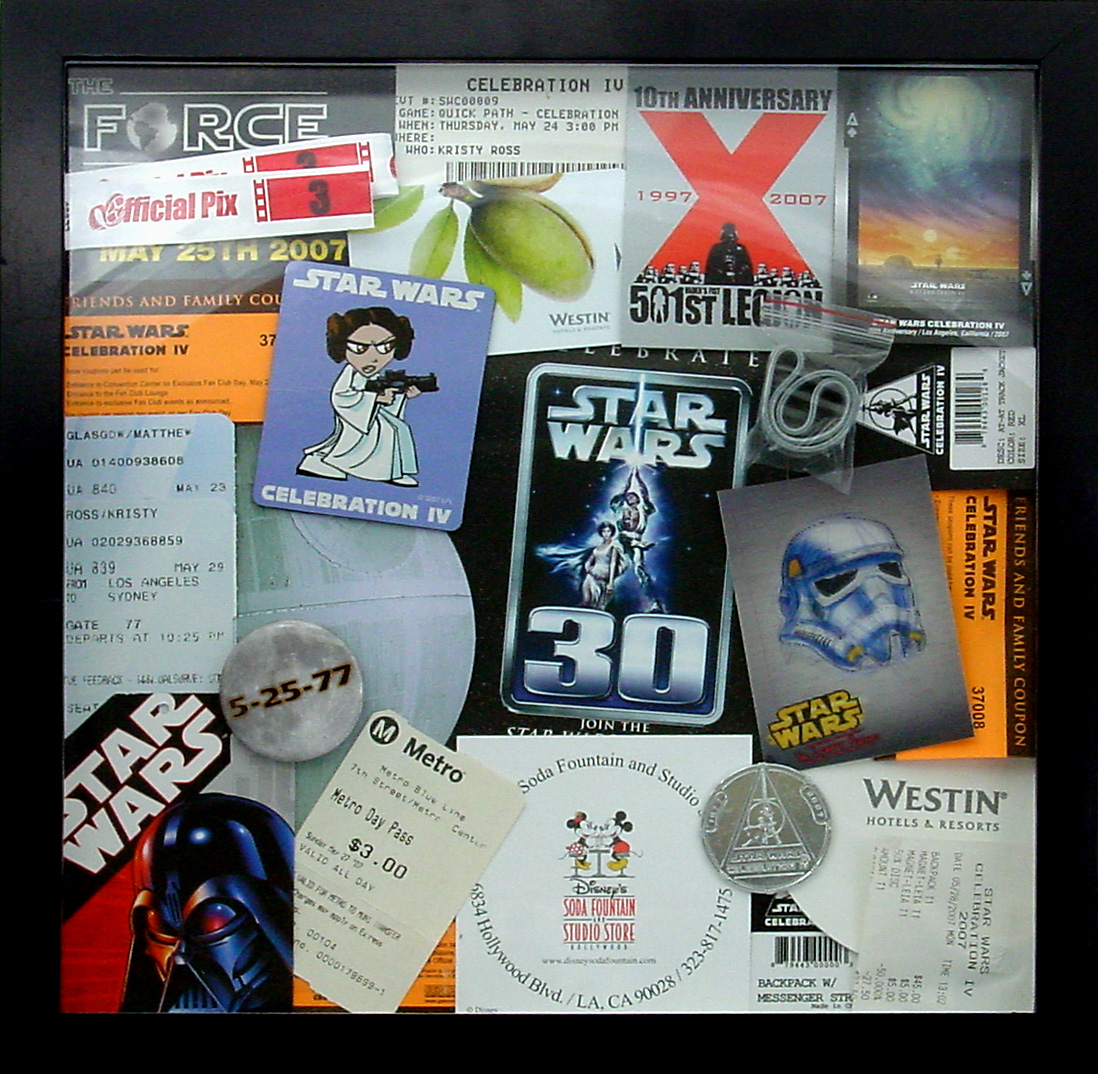This detailed image is a screenshot capturing a collage of Star Wars memorabilia displayed within a black-framed picture frame. Dominating the scene is an array of collectible items, including ticket stubs, advertisements, and anniversary memorabilia chronicling various Star Wars events and milestones. An adorable cartoon image of Princess Leia wielding a laser pistol is featured prominently on a cardboard cutout from Star Wars Celebration IV. In the bottom right corner, an image of Darth Vader’s helmet stands out aggressively beneath the Star Wars logo. A Disney-themed item showcases Mickey and Minnie Mouse sharing a soda, hinting at a Hollywood Boulevard soda fountain and studio store, likely connecting to Disney's Star Wars attractions. A coin referencing the "A New Hope" poster is meticulously engraved, while above it, the New Hope logo highlights what appears to be a 30th Anniversary celebration. The composition also includes a 10th anniversary badge for the 501st Legion, vintage movie posters—most notably a classic "A New Hope" scene with Luke Skywalker hoisting his lightsaber alongside Princess Leia—, and a Metro Day Pass and various pieces of paper, Metro cards, and advertisements. The entire collage gleams with iconic Star Wars imagery, featuring characters like Leia, Darth Vader, and Stormtroopers set against backdrops of red, black, and green hues.